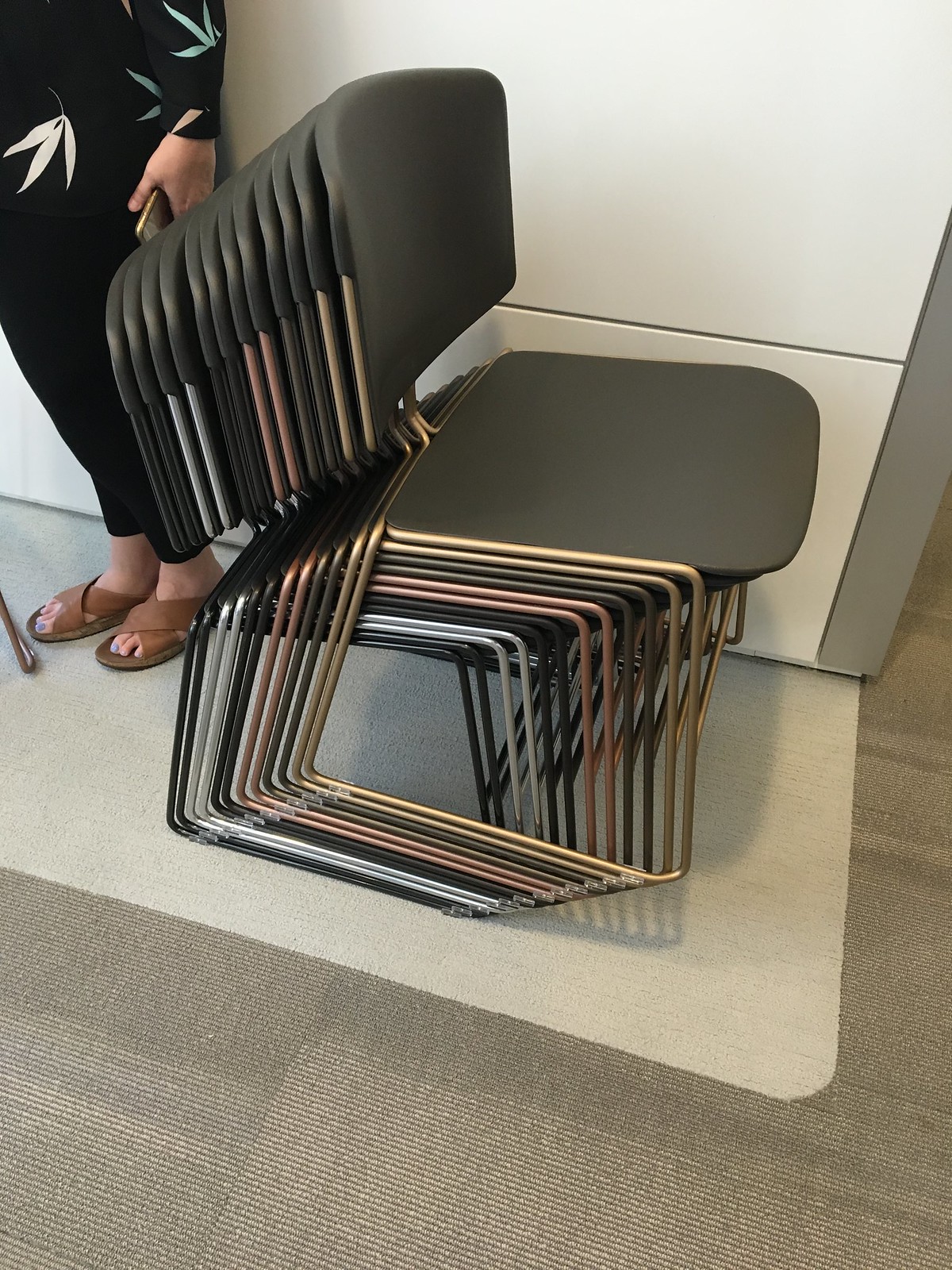This photograph showcases a stack of 12 to 13 chairs neatly arranged in a room with a gray and white carpet. The chairs, typically found in office or convention settings, feature black plastic seats and backrests, with metal frames that vary in color—gold, bronze, silver, black, and even a pink hue. The frames are designed with wire loops that provide support and allow the chairs to stack snugly, slightly angling upward and forward from the bottom to the top. Alongside the stacked chairs, on the left, stands a woman partially visible. She is wearing brown crisscross sandals showcasing her lavender-blue painted toenails, black pants, and a black sweater adorned with white and blue leaf patterns. She holds a smartphone in her left hand. The setting includes a juxtaposition of a thicker gray carpet and a lighter, possibly beige, carpet strip next to a white wall.